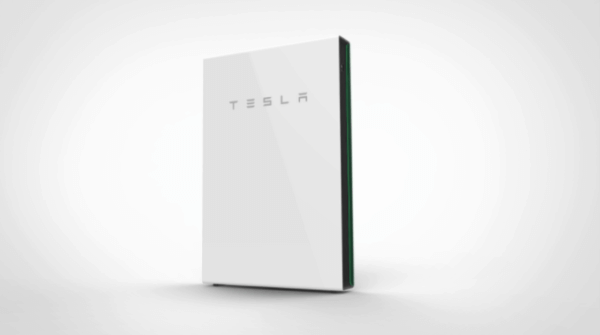The image is a wide rectangle with dimensions approximately twice as wide as it is tall, set against a light gray background. Centered in the composition is a tall rectangular object resembling a monolith but shaped like a book, although it is not an actual book. This object features a light gray cover that gradients to a slightly darker gray towards the left edge, which is itself darker than the background.

The right-hand edge of the object is about an inch thick and is colored black. The cover features the word "Tesla" written in the distinctive style of the Tesla logo, in a medium gray tone that contrasts subtly with the cover's lighter shade. The object appears to rest on a surface that seamlessly blends with the background, making it difficult to discern any definitive edges. There is a slight shadow beneath the object, extending faintly to both the left and right sides. Additionally, a thin, green vertical line runs along the entire height of the black right-hand edge of the object, adding a subtle pop of color to the otherwise monochromatic palette.